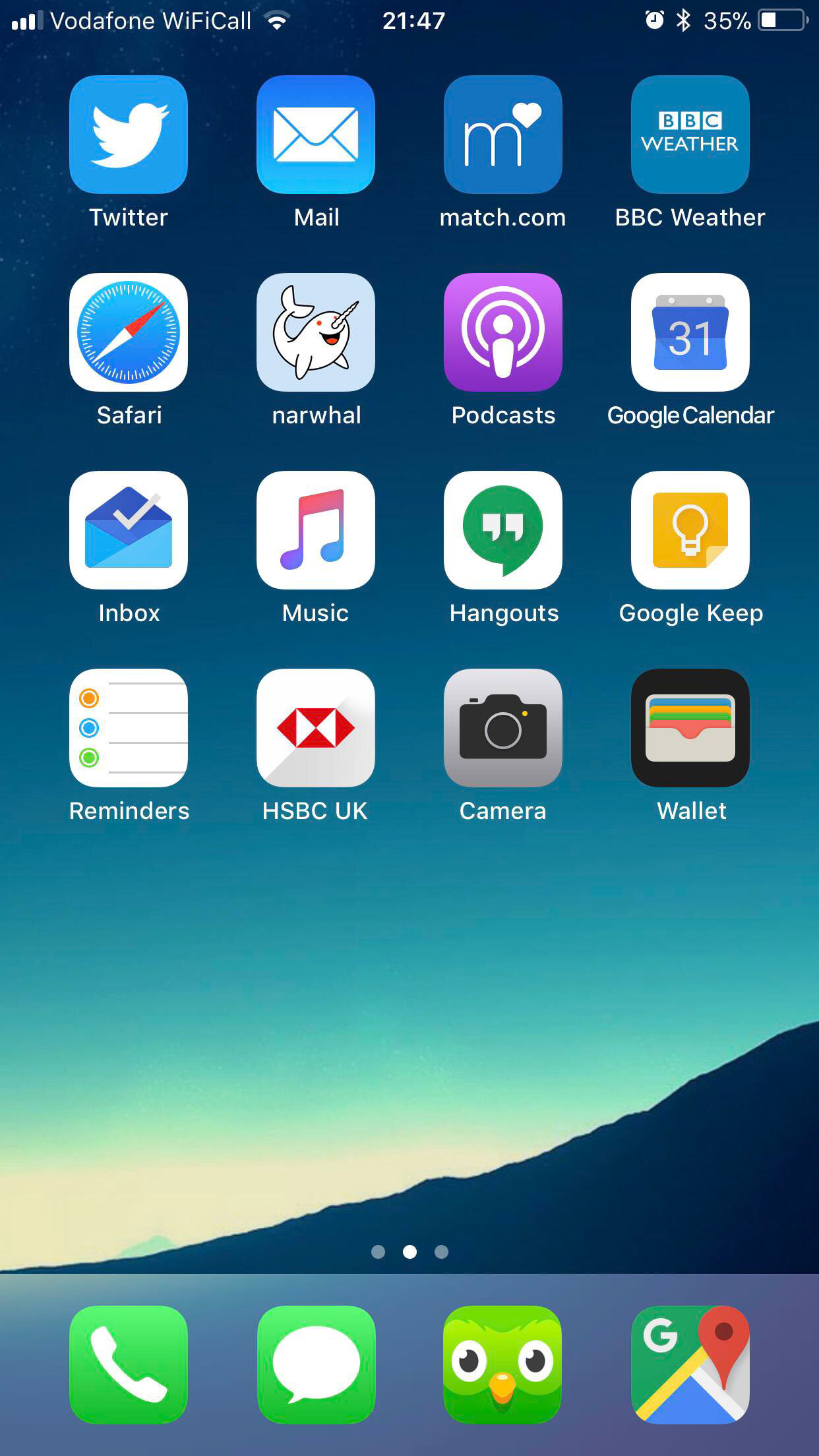This screenshot showcases a smartphone home screen set against a serene and picturesque background of a sunset scene. The backdrop features a dark blue sky, adorned with sparkling stars on the left side, casting an evening ambiance. Dominating the lower right corner, a dark blue landmass, possibly a hill or mountain, adds depth to the image. Behind this land formation, sun rays in shades of pink and yellow peek through, gradually lightening the surrounding sky and creating a captivating blend of colors.

The home screen is populated with a variety of app icons, showcasing a diverse range of functionalities. From left to right, these include Twitter, Mail, Match.com, BBC Weather, Safari, Narwhal, Podcasts, Google Calendar, Inbox, Music, Hangouts, Google Keep, Reminders, HSBC UK, Camera, and Wallet.

At the bottom of the screenshot, a bluish-gray border, presumably indicating the most frequently used apps, houses four key icons. On the far left is the green Phone icon, followed by the Messaging app. Next is the Duolingo app, identifiable by its distinctive green owl face. Lastly, on the far right, sits the Google Maps icon, completing the array of essential applications.